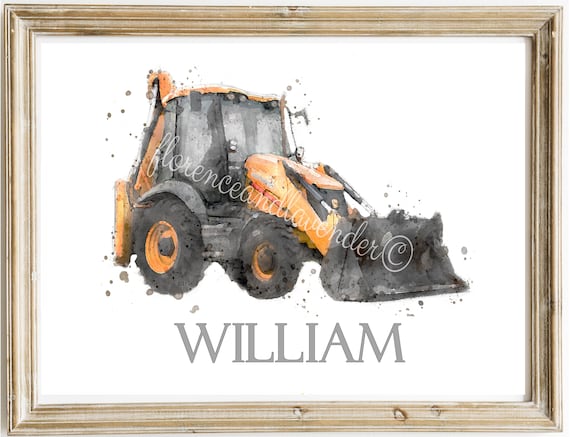This is an image of a watercolor painting of a bulldozer, elegantly framed in a light tan wooden frame adorned with prominent knots outlined in black, giving it a rustic character. The bulldozer depicted in the painting has a cab made completely of light black, smoked glass, providing a somewhat opaque view inside. It features a yellow roof and a series of four lights positioned above the windshield. The machine has a front bucket painted black, ideal for scooping dirt or concrete, attached to yellow metal forks with visible black hydraulic cylinders. The vehicle sports both front and back buckets, hinting at its multifunctional design, with small black front wheels and larger rear ones, possibly denoting a backhoe loader. Surrounding the bulldozer in the painting, there are specks of color resembling dirt, adding to the realistic portrayal of a work environment. Above the painting, penned in cursive writing, are the words "Florence and Lavender" accompanied by a circled 'C'. A peculiar but striking addition is the name "William" inscribed in gray at the base of the image. The unique combination of these detailed elements encapsulates a blend of technical precision and artistic elegance.